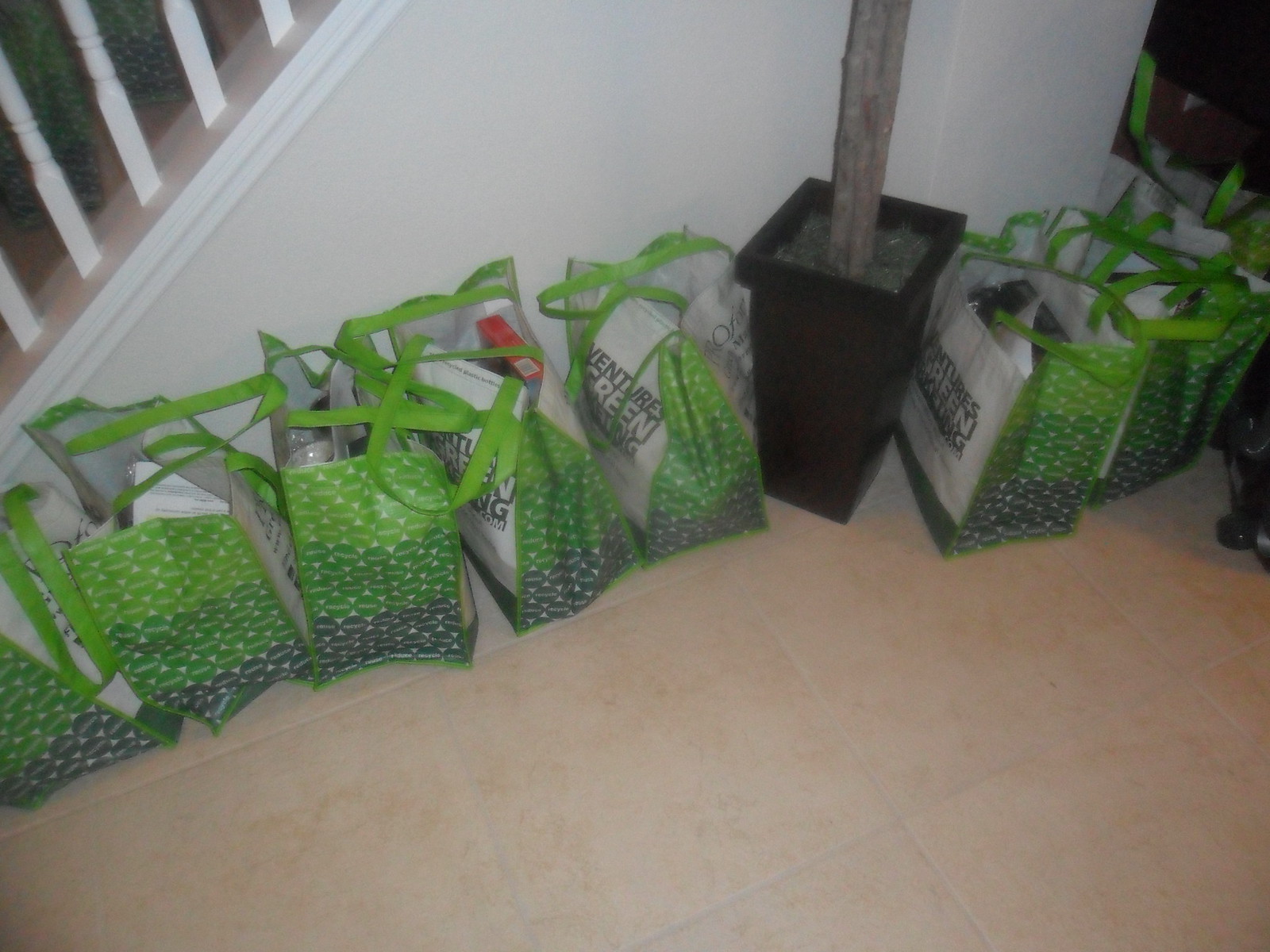The photograph captures an indoor scene featuring a staircase with white banisters ascending alongside a white wall. Below, a slightly salmon-colored tiled floor adds warmth to the space. Positioned against the staircase is a row of seven or eight translucent green shopping bags, gradients ranging from leaf green to hunter green, each with a white panel on the front displaying illegible text, including "Ventures Green" and a web address. These reusable bags, patterned and durable with long fabric handles, appear to contain various food items, one visibly holding a red box resembling a package of pasta or a cake. Nestled among the bags is a slender tree growing in a tall, black flower pot, displaying only its skinny wooden trunk amidst the scene.